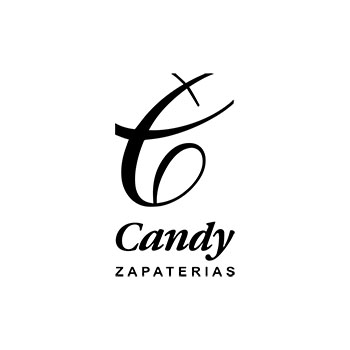The image features a minimalistic yet stylish company logo against a solid white background. The centerpiece of the logo is a large, black cursive letter "C," partially cut off at both the top right and top left sections, giving it an abstract appearance. Below this fancy "C," the word "Candy" is prominently displayed in a bold, italicized black font, with only the "C" capitalized and the rest of the letters in lowercase. Directly underneath "Candy" is the word "ZAPATERIAS," written in a smaller, all-uppercase black font. The simplicity of the black text against the white backdrop gives the logo a clean, modern look.